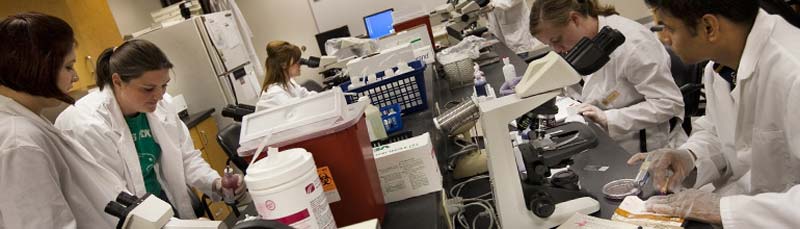The image depicts a laboratory scene where six medical professionals, including at least three women and one man, are engaged in intensive research. They are all dressed in white lab coats and plastic gloves, indicating a sterile environment. One woman is distinguishable by her green shirt with white lettering underneath her coat. The individuals are positioned around desks that are seamlessly joined together, creating a workbench filled with scientific equipment. This includes several microscopes in use, petri dishes, and various containers—some specifically identified as white with red labeling and another red container with an orange and white label, which might be for blood. A white refrigerator stands in the left corner of the room, contributing to the clinical setting.

Computer monitors with blue screens and white icons are visible along the upper part of the image. Baskets holding supplies like bottles, cleaners, and potentially hazardous disposal bags are scattered across the desks. The setting is well-lit, with prominent colors like red, white, green, blue, black, yellow, and a hint of gold. The image's panoramic nature captures a broad view but cuts off some details at the bottom. Notably, one person’s head is cropped out, rendering their gender indistinguishable. This detailed scene highly suggests a hospital or laboratory where medical research, likely on germs or chemicals, is being conducted.